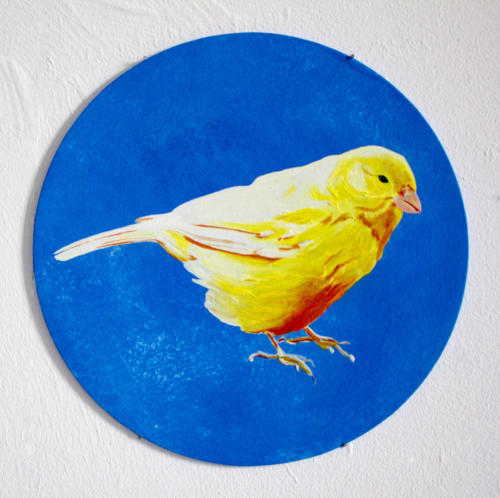The image depicts a meticulously detailed painting of a yellow bird, accented with white and dark orange textures, facing to the right with its head leaning slightly forward and its gaze directed downward. With black eyes and an orange beak, the bird showcases a gradient where its yellow feathers subtly blend into white on its back and belly. Both of its feet are visible, standing against an undefined backdrop, and its wings are held close to its body. A small tail extends slightly from the left side toward the back. The painting is encapsulated within a round blue background that features varying tones, from darker shades in the bottom right and top areas to lighter sections with specks of white in the bottom left. This blue circle is centered on a white textured surface, and the entire composition is perfectly symmetrical, emphasizing the delicate details of the bird against the contrasting background.